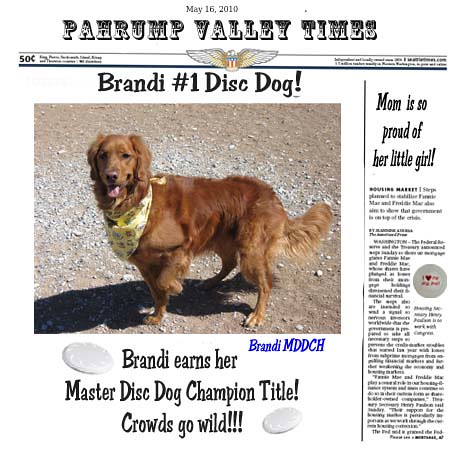This image is a vibrant front page of the Pahrump Valley Times from May 16, 2010, featuring a joyous occasion for dog enthusiasts. The headline reads "Brandy No. 1 Disc Dog!" above a captivating color photograph of Brandy, a reddish-gold golden retriever adorned with a yellow kerchief around her neck, happily looking at the camera. The photograph, set against a concrete ground, showcases Brandy as she proudly earns her Master Disc Dog Champion (MDDCH) title. The caption beneath the photo proudly exclaims, "Brandy Earns Her Master Disc Dog Champion Title! Crowds Go Wild!" Flanking the main photo are images of two white disc dog discs, emphasizing her achievement. To the right of the main feature, a vertical article with the headline, "Mom Is So Proud of Her Little Girl!" details the emotional journey and pride Brandy’s owner feels about her triumph in the tournament. At the very top of the page, the newspaper’s masthead, embellished with an eagle emblem in red, white, and blue, prominently displays "Pahrump Valley Times" along with the date and a price tag of 50 cents. This colorful and detailed presentation celebrates Brandy's remarkable accomplishment, capturing the essence of community pride and canine excellence.